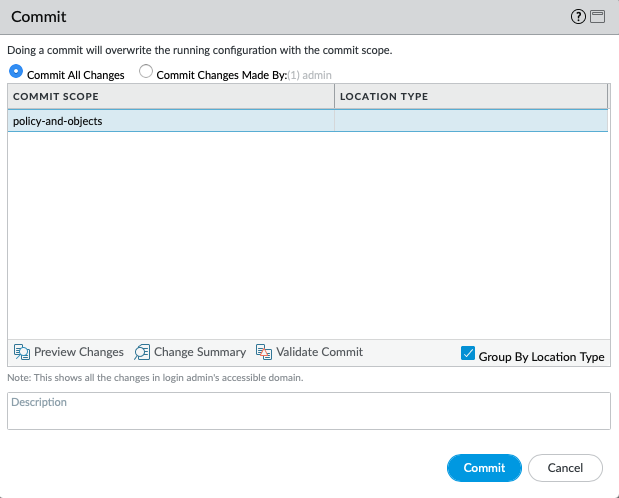The image displays a rectangular interface screen that is wider than it is tall, with a width approximately 20% greater than its height. There is a gray header bar at the top, featuring the term "commit" on the upper left corner, a question mark enclosed within a circle, and a window icon on the upper right side.

Below the header, aligned to the left, a message states: "Doing a commit will overwrite the running configuration with the commit scope." This indicates that the interface pertains to the commit section of an application.

Further down, there are two selectable options represented by radio buttons. The first option, which is selected and filled in blue, reads "Commit all changes." The second option, unselected and empty, reads "Commit changes made by" followed by a colon and the phrase "(1 admin)" in faint gray text, suggesting it pertains to a specific user.

Underneath these options is an empty chart with the title "Commit Scope." The chart is divided into two sections, with "location type" appearing on the right side. There is one entry within the chart, highlighted and indicating it is selected. The entry reads "policy and objects," with a highlight strip spanning from the left to the right side of the interface, emphasizing this row.